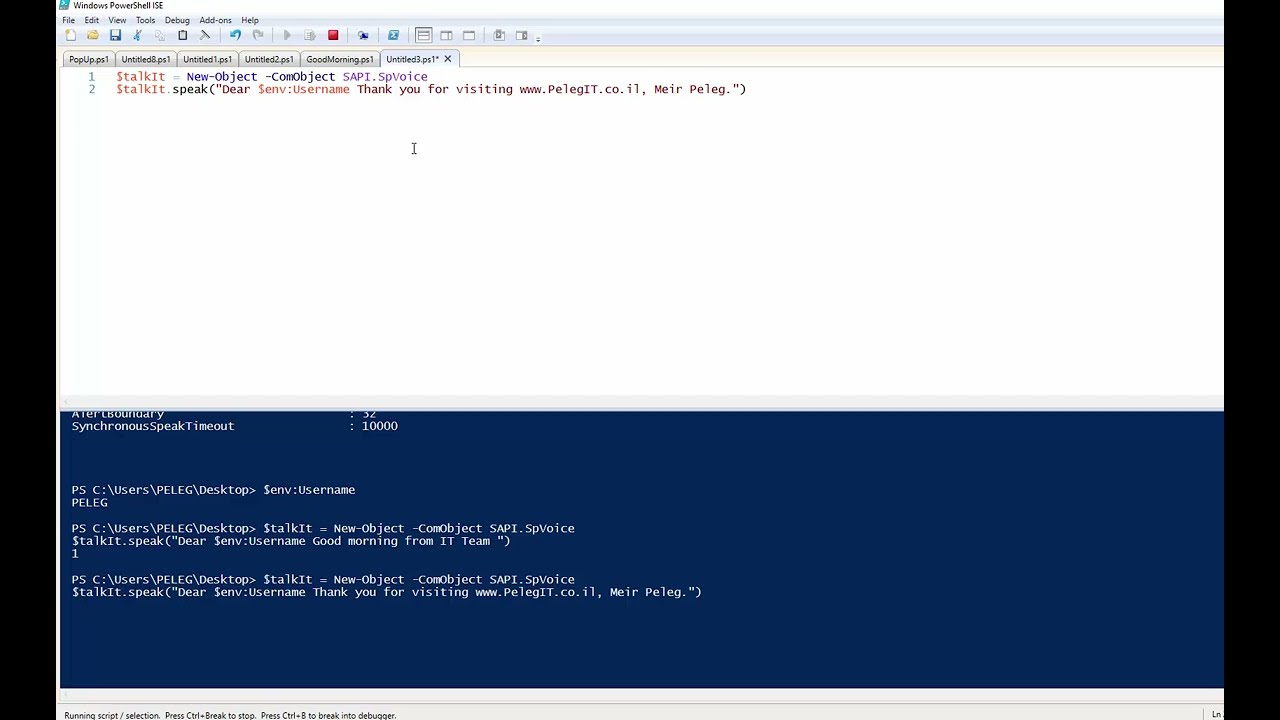The image is a horizontal rectangular screenshot from a computer screen, showcasing a piece of code. At the top, there is a navigation bar with buttons like file and save, followed by a row of tabs labeled "popup.ps1," "untitled1," "untitled2," "untitled3," and "good morning." The upper half of the screen displays code against a white background in red, blue, and black text. Lines of code feature instructions for creating and using a style kit object and include details like user paths and messages. The text includes terms such as "new object," URLs, and repeated references to the user "peleg" and style kits. The lower half of the screen transitions to a dark blue background with white text, continuing the code with syntax involving user paths and actions. The visual style of the screenshot is realistic and detailed, mimicking the look of a freeze-frame photograph of an active computer monitor.